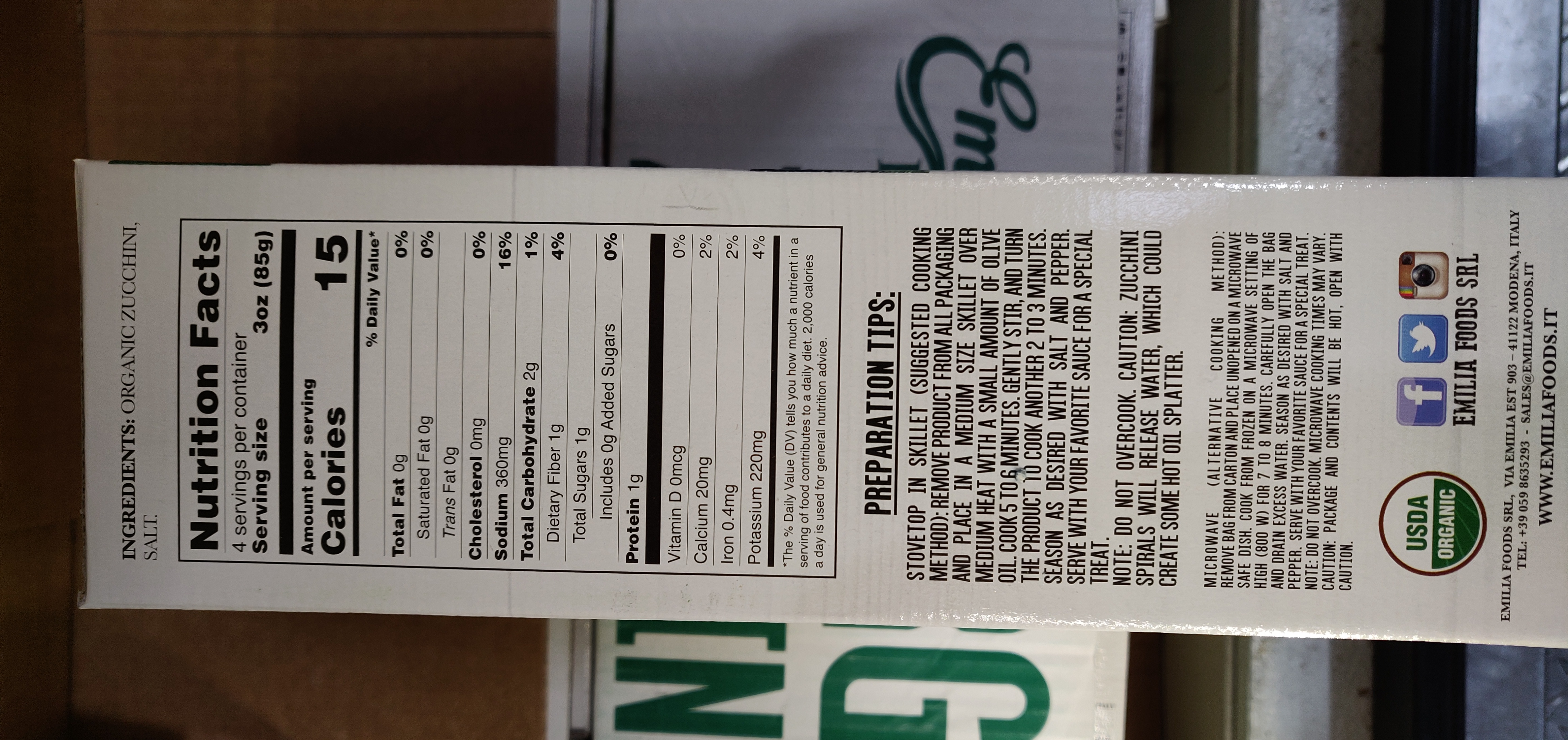The image displays the side panel of a food box, which appears rotated to the left. At the top, the ingredients list prominently features organic zucchini and salt. Below this, the nutritional facts are detailed: a serving size of three ounces contains 15 calories, zero grams of total fat, saturated fat, and trans fat, 360 milligrams of sodium (16% of daily value), two grams of total carbohydrates (1% daily value), one gram of dietary fiber (4% daily value), one gram of total sugars with no added sugars, and one gram of protein. Additionally, it lists 20 milligrams of calcium, 0.4 milligrams of iron, and 220 milligrams of potassium (4% daily value).

Further down, the box provides cooking instructions, with stovetop and skillet methods detailed first and a microwave option suggested in smaller print as a less preferred method. The bottom of the side panel features a green and white USDA Organic logo enclosed in a circle and social media icons for Facebook, Twitter, and Instagram, linked to the brand Amelia Foods.